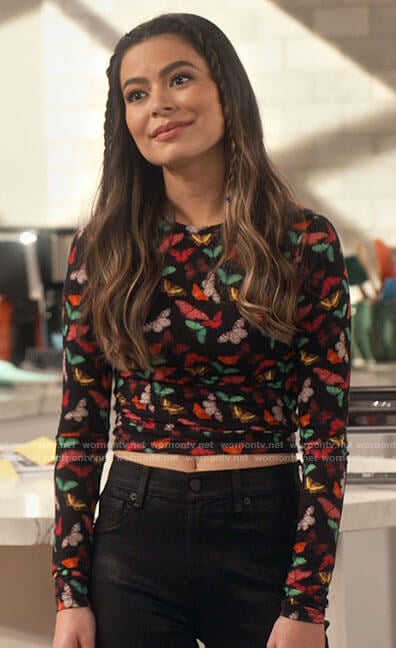The image captures a teenage girl, resembling the celebrity Miranda Cosgrove, positioned perfectly in the center of a kitchen scene, likely on the set of a TV show. The setting features blurred background elements including a kitchen island, a coffee maker, and a utensil container. The girl, with a Caucasian complexion and medium-length brown hair styled with two front braids, gazes slightly over the left shoulder of the camera with a slight tilt to her head and a partial smile. She wears makeup, including lipstick and eyeliner, and sports a long-sleeved black shirt adorned with colorful butterflies, revealing her belly button, paired with black jeans. The color palette of the image includes shades of yellow, brown, olive, pink, white, green, blue, and black.